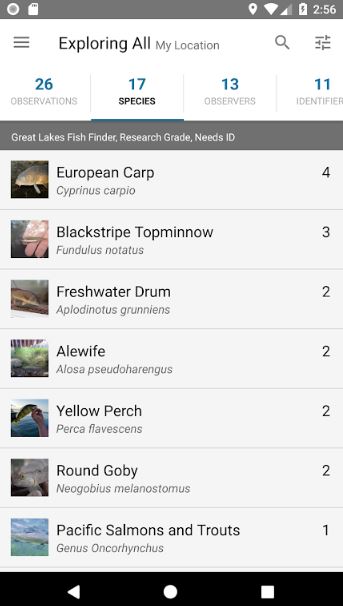A mobile phone screen displaying a fish identification app is shown in this image. The top-left corner features several icons: a circle with a filled-in circle inside, a piece of paper with a folded corner, and a map pin. On the right are the Wi-Fi signal, a full battery icon, and the time '2:56' (unclear if it's a.m. or p.m.). Below these are three lines indicating a menu bar, and the text "Exploring" followed by "My Location." 

A search bar is prominently displayed, accompanied by a line with a small tack icon. The interface specifies "26 observations" in aqua blue text. The text "Observations," "26 Observations," "17 Species," "13 Observers," and "11 Identifiers" are also displayed, with "Species" in black to highlight the currently selected category. All these labels are capitalized for emphasis.

Beneath this is a dark gray rectangle with white text stating, "Great Lakes Fish Finder Research Grade Needs ID." The listed species include:
- European Carp (4 observations)
- Blackstripe Topminnow (3 observations)
- Freshwater Drum (2 observations)
- Alewife (2 observations)
- Yellow Perch (2 observations)
- Round Goby (2 observations)
- Pacific Salmons and Trouts (1 observation)

Each species is accompanied by an image to the left, aiding in visual identification. At the bottom of the screen, navigation buttons are displayed on a black rectangle: a left-pointing triangle, a circular button in the middle, and a square, all in white.

This detailed layout helps users identify and catalog various fish species efficiently.